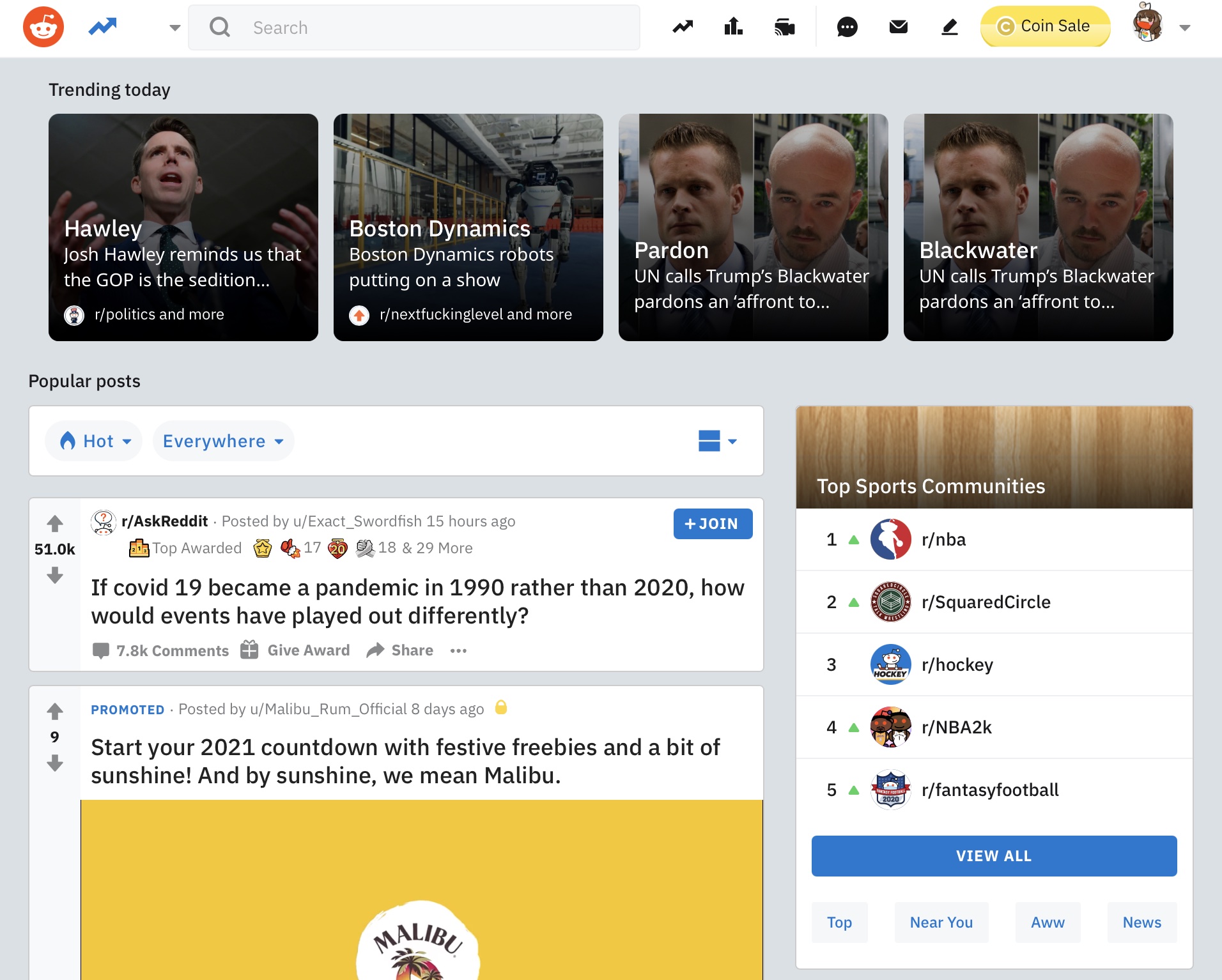A detailed screenshot of the Reddit homepage showcases various elements at the top, beginning with the Reddit logo, followed by the blue "Trending" tab. Next to this is the search bar along with several other navigation tabs including Trending, Popular, Videos, Messages, Notifications, and Posts. Additionally, there is a prominent blue button for a coin sale and the user's profile icon.

Beneath this navigational bar, the "Trending Articles" section is visible, featuring topics such as "Holly," "Boston Dynamics' robot show," and "UN calls Trump's Blackwater pardons an affront." The "Blackwater" article appears twice, accompanied by the same image of two men, although the latter portion of the title is cut off.

Further down, the "Popular Posts" section can be seen, highlighting posts that are currently hot and trending. The top post is from r/AskReddit, posing the question: "If COVID-19 became a pandemic in 1990 rather than 2020, how would events have played out differently?" This post has garnered 51,000 interactions and 7.8k comments. Below this, there is a promoted post for Malibu Algonquin.

On the right side of the screen, a column dedicated to top sports communities is displayed, listing NBA Circle, /r/squarecircle (wrestling), Hockey, NBA 2K, and Fantasy Football among the highlighted subreddits.